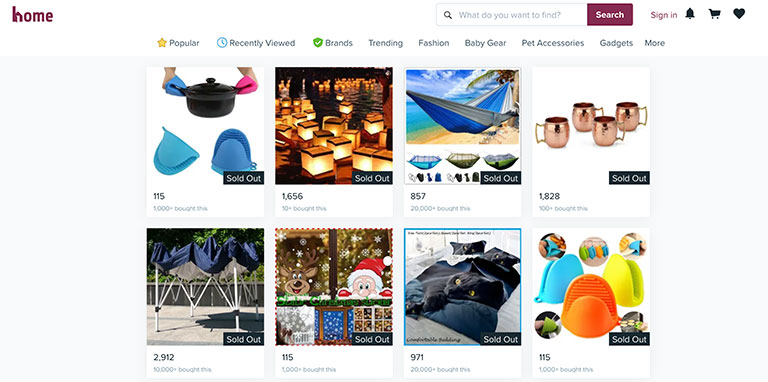Screenshot of an E-Commerce Website Interface:

The screenshot captures the homepage of an e-commerce website featuring a variety of items for sale. In the top left corner, the word "Home" is prominently displayed, indicating the main navigation link. Moving right across the top bar, there is a search button accompanied by a search field, allowing users to easily find specific products. Further along the top bar, options to "Sign In," a notification bell icon, a shopping cart icon, and a heart icon for wishlist items are visible.

Below this main navigation bar, a secondary menu offers additional categories including “Popular,” “Recently Viewed,” “Brands,” “Trending,” “Fashion,” “Baby Gear,” “Pet Accessories,” “Gadgets,” and a “More” button for extra options.

Beneath this secondary menu, a grid of tiles showcases various products available on the website, some of which are currently sold out. The items featured in these tiles include: 

- Oven gloves made of rubber
- Square storage cubes
- A hammock
- Golden goblets
- A foldable camping chair
- Christmas window decorations
- A black kitten
- A black duvet set
- Unique rubber oven mitts designed to look like animal mouths

Each product tile provides a visual representation of the items, giving users an idea of what to expect when browsing through the website.